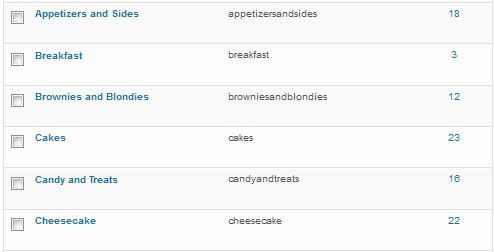**Detailed Caption:**
The image depicts a landscape-oriented screenshot of what appears to be a restaurant inventory tracking application. The interface consists of a list categorized by various food items, each delineated by thin gray horizontal lines. Each category name is highlighted in a teal font, while the accompanying text and numbers are in either dark gray or black font for clarity. 

The layout comprises a series of checkboxes aligned to the left of each category name, although none of the boxes are currently checked. The categories and their respective counts are organized in two columns:

1. **Appetizers and Sides**: Count – 18
2. **Breakfast**: Count – 3
3. **Brownies and Blondies**: Count – 12
4. **Cakes**: Count – 23
5. **Candies and Treats**: Count – 16
6. **Cheesecake**: Count – 22

Additionally, each row features the category name duplicated in the adjacent column but presented as a continuous text string without spaces. This meticulous arrangement helps keep the information structured and quickly accessible, providing a concise overview of the inventory for easy tracking and management.